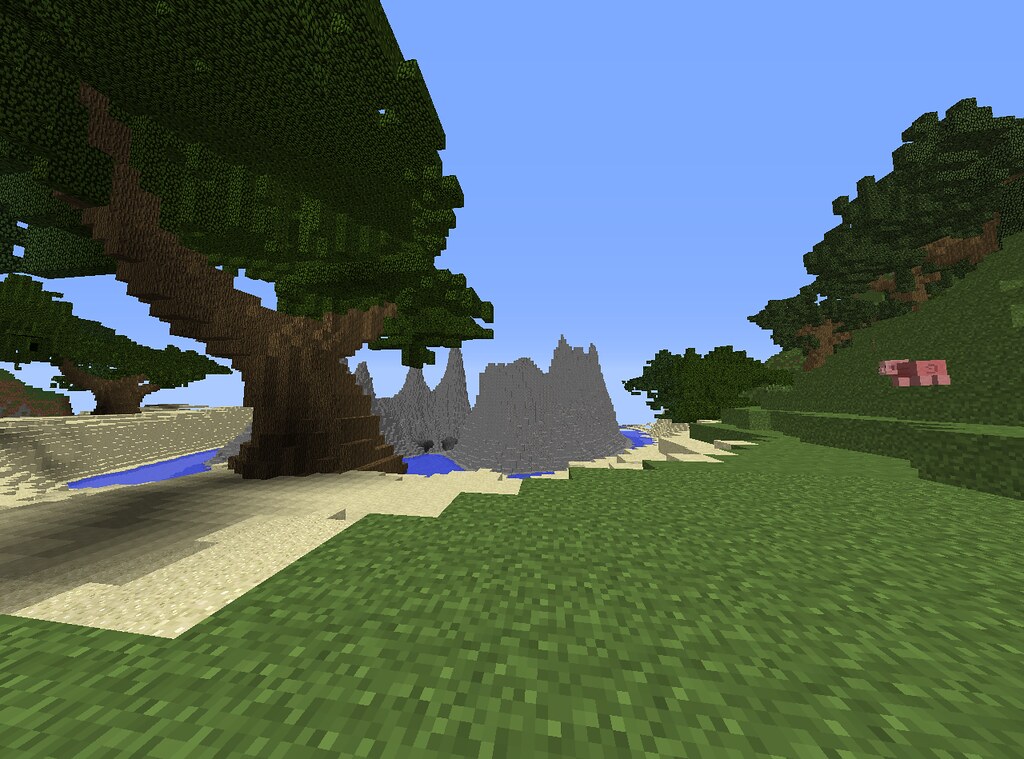In this Minecraft scene, an expansive sandy desert stretches across the foreground, composed of numerous sand blocks. Adjacent to the sand, a vibrant blue body of water adds a contrasting splash of color. At the horizon, stone mounds punctuate the landscape, providing a rugged backdrop. To the right, green blocks are intricately stacked, forming the foundations of trees. On the left side of the image, wooden blocks ascend, leading up to a canopy of dense green foliage, resembling the treetops. The far left background showcases additional trees under a clear blue sky, framing the serene setting. Dominating the right side of the image, a charming Minecraft pig, crafted from paper cubes, adds a whimsical and playful touch to the otherwise naturalistic environment.